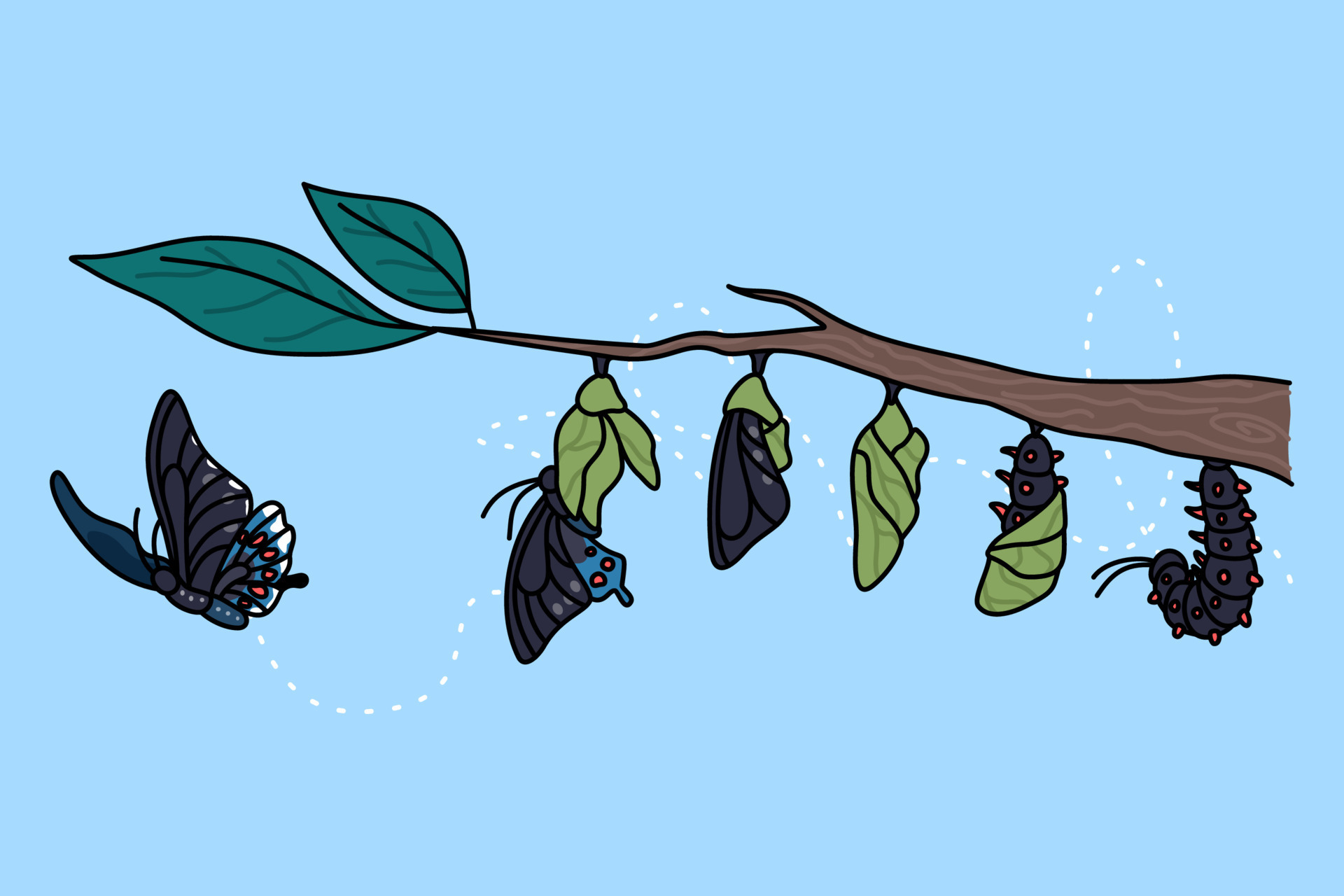The illustration captures the detailed maturation process of a caterpillar transforming into a butterfly, depicted in a series of sequential stages from right to left. Set against a light blue background suggesting the sky, the tree branch in the image is simple, with two green leaves on the left end, one slightly larger than the other. The stages begin with a black caterpillar with red feet hanging upside down from the branch. Sequentially to the left, the caterpillar is then shown half-hidden in a green cocoon. Following this, the caterpillar is fully encased in the green cocoon. In the subsequent stages, the cocoon begins to open, revealing a butterfly with predominantly black wings, accented by patches of dark blue, white, and pink. By the final stage, the butterfly is completely free and in flight. Connecting each stage is a white dotted line, emphasizing the process of metamorphosis. The overall style is cartoonish and quick, adding a simplistic yet informative charm. There is no text in the illustration.